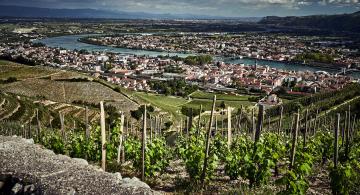This vivid photograph captures a picturesque landscape, possibly situated in a small town or a remote area, reminiscent of regions in Italy or Thailand. In the immediate foreground, neat rows of plants, resembling a vineyard or perhaps tomato plants, stretch across green fields. The fields gently slope downhill towards a tranquil, curving river. Along the riverbank, a collection of approximately 200 houses with reddish-brown roofs and white walls creates a charming, cohesive appearance, evoking the architectural styles of Spanish or Hispanic settings. In the distant background, a majestic mountain ridge is silhouetted against a deep blue sky. The scene is partially framed by a diagonal section of a stone wall in the bottom left corner, adding a textured element to this serene and extensively detailed landscape.